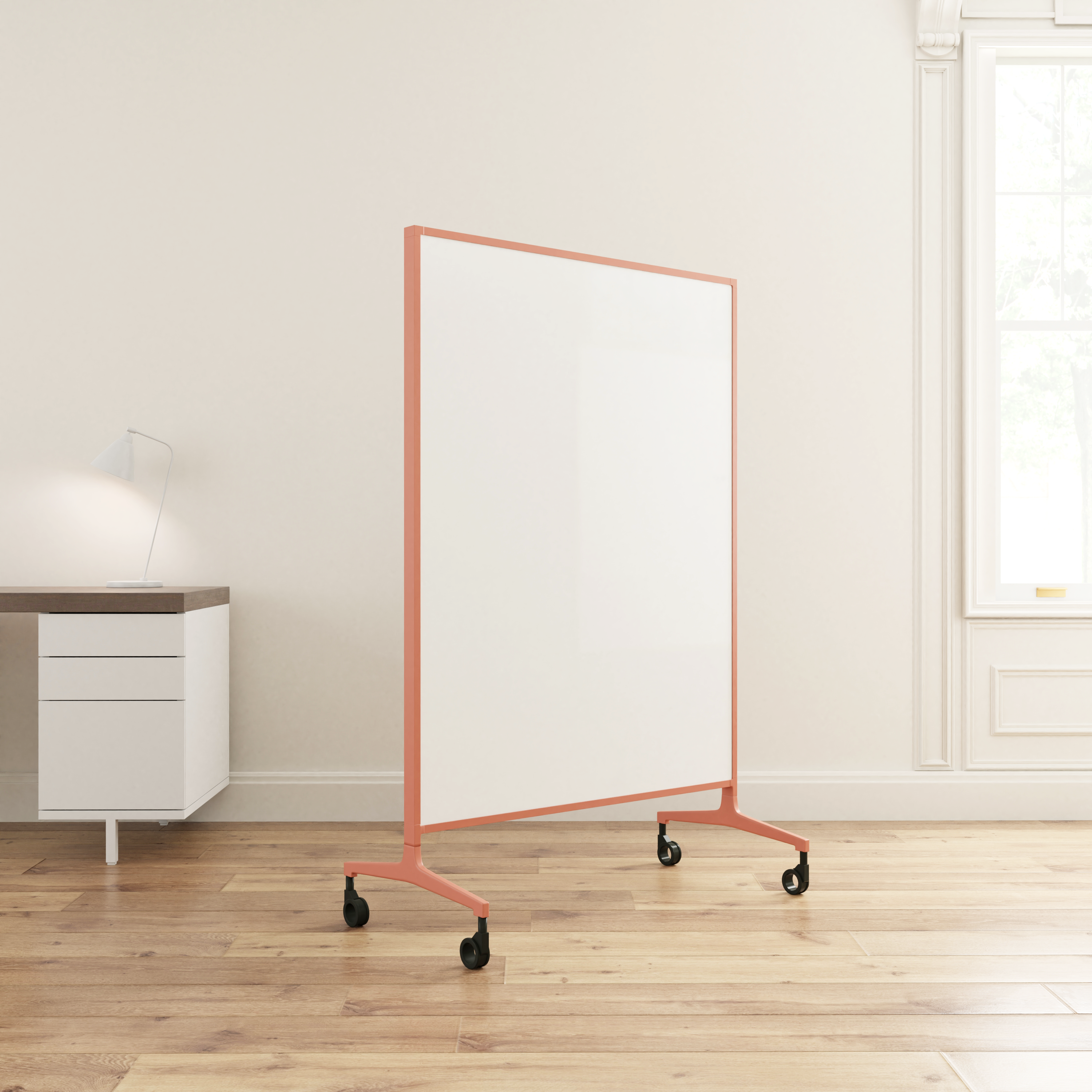This image showcases a clean, neutral-colored room with a large, mobile panel mirror at its center. The mirror, framed in a salmon-colored metal, stands on four black wheels, allowing it to be easily moved around the space. The room features cream-colored walls and a light pine-colored plank wood floor. To the left, partially in view, is a white desk with a dark wooden top supporting a wire-type desk lamp. On the right side of the image, a large picture window with wainscot molding beneath it lets in natural light. The overall ambiance of the room is minimalistic and tidy, highlighting the central feature of the rolling mirror.